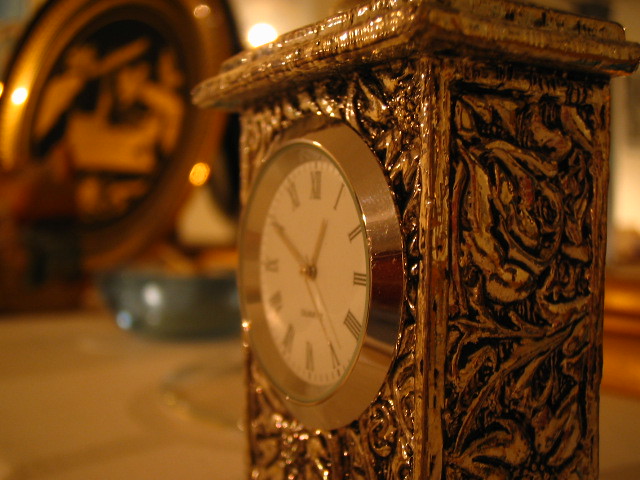This image captures an elaborate mantel clock with a gold-toned finish, prominently positioned so that the front right-hand corner is nearest to the camera. The clock's design is intricate with deeply engraved floral patterns, including roses and leaves, which are accentuated by dark, almost black recesses. The clock features a white face adorned with gold Roman numerals from 1 to 12, encompassed by a thick, gold border exhibiting signs of wear. The hour, minute, and second hands are gold in color. Although the background is blurred, it suggests a sophisticated setting with a blue, possibly clear bowl or ashtray, and a framed piece of art with a round, oval shape that appears to have a decorative design. The ambient lighting hints at an indoor scene, possibly illuminated by artificial light, adding to the antique and elegant atmosphere.